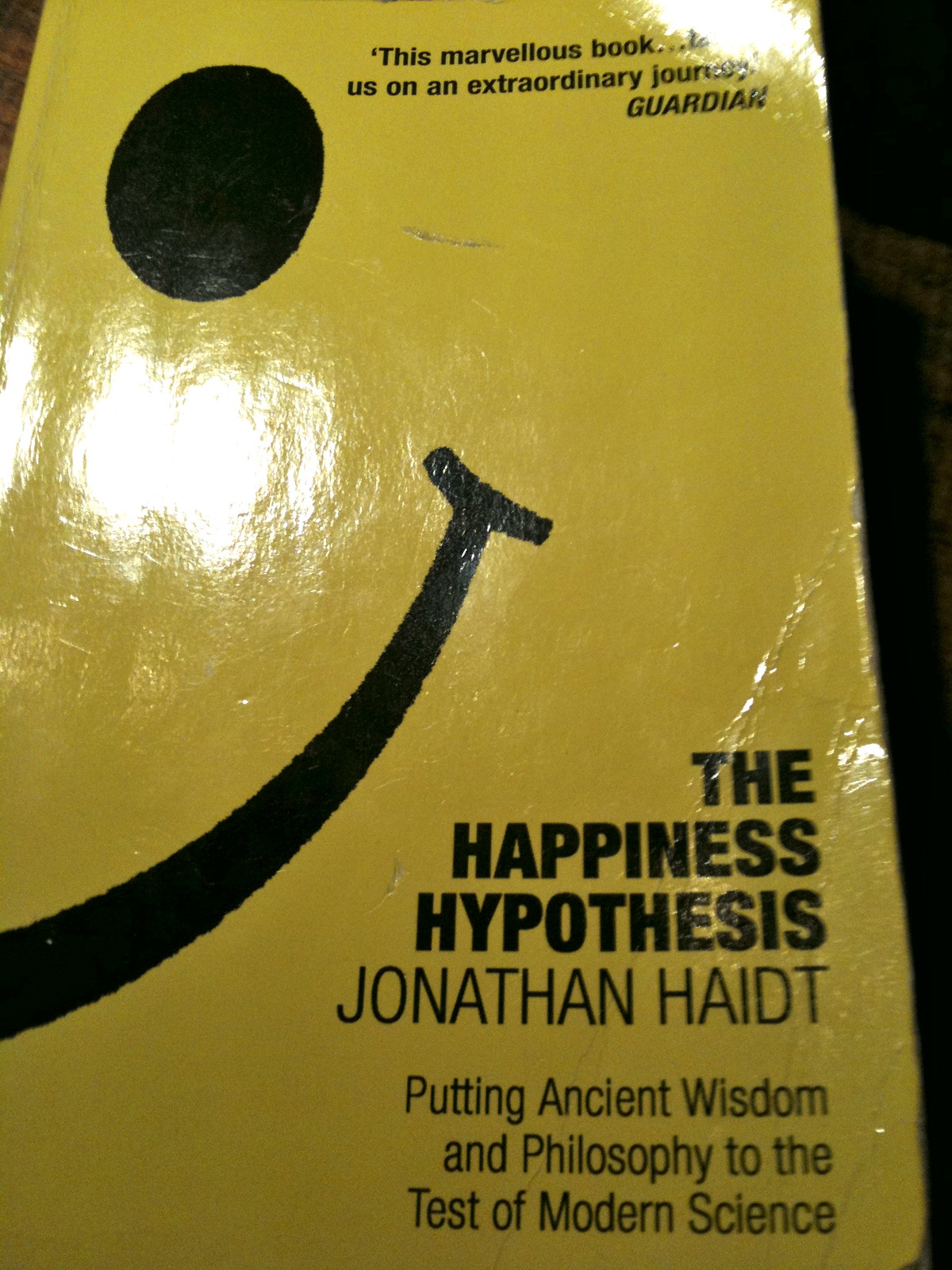The image depicts a close-up photograph of the cover of a paperback book set against a black background, making the setting unidentifiable. The book cover is predominantly yellow and features a glossy, reflective finish that catches the light. The cover displays half of a stereotypical simplified smiley face, with a black oval for an eye above a curved line, positioned on the left half. The other half of the face likely appears on the back cover of the book. The title and author details are printed in black text on the right side, with the top right corner reading "This Marvelous Book, Us on an Extraordinary Journey, Guardian." Below this, in a larger font, the title "The Happiness Hypothesis" is presented, followed by "Jonathan Haidt, Putting Ancient Wisdom and Philosophy to the Test of Modern Science" in a smaller font at the bottom right. The book's positioning and the photograph's composition suggest a casual snapshot taken in a dark room, emphasizing the book's shiny cover.